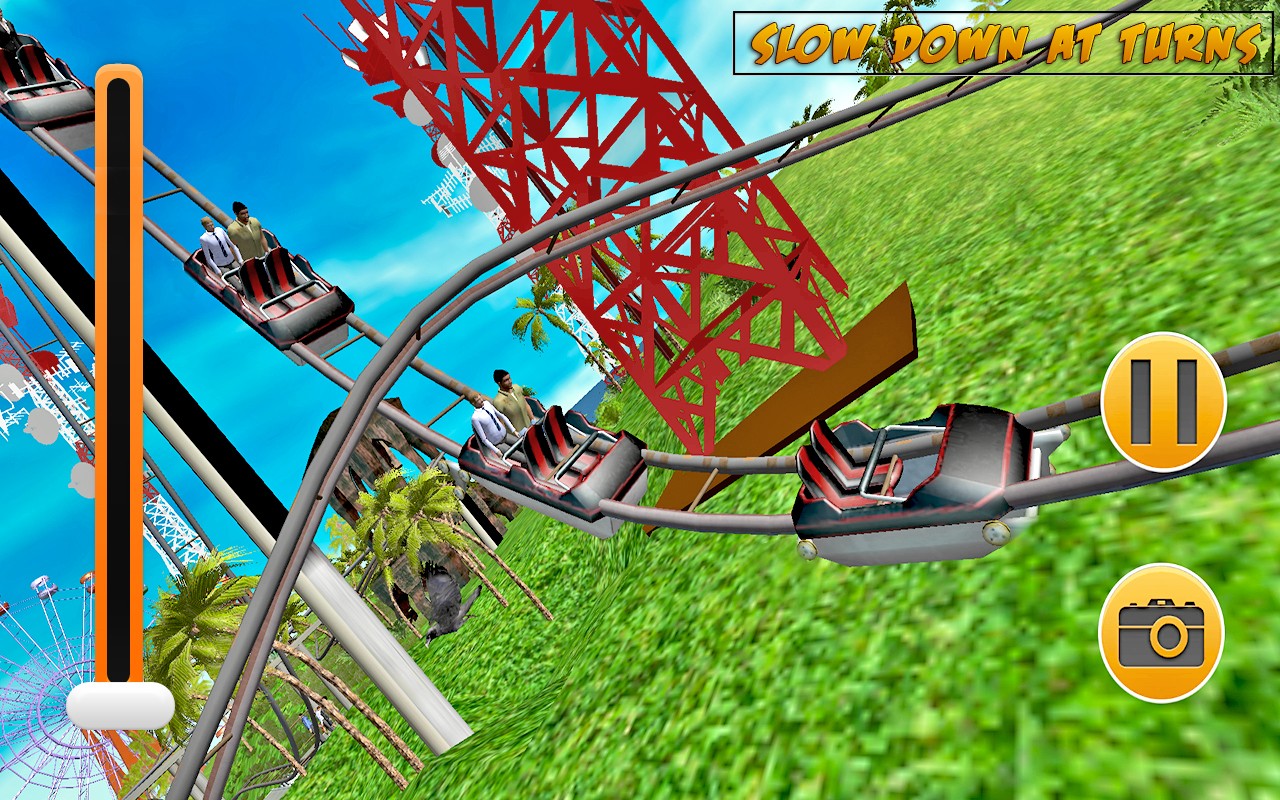This is a screenshot from a mid-2000s simulation game, likely a theme park or roller coaster game. The scene is set in an outdoor environment featuring a roller coaster with a computer-generated, somewhat dated aesthetic. The roller coaster has a steeply descending black track with four visible cars. The first and the last cars are empty, while the middle two cars each have two identical-looking passengers. 

In the second car, there is a man wearing a long-sleeve white shirt with a tie on the left, and a man in a light yellowish shirt on the right. The third car has at least one man dressed in black. To the right of the track, yellow circles display a pause symbol and a camera icon. 

In the background, you can see green grass, some palm trees, a water body, and a blue sky. There's also a red metal tower behind the roller coaster and another section of the track curving above. A yellow sign at the top right corner reads "slow down at turns" in a cartoony font. In the bottom left corner, a Ferris wheel is partially visible. To the left of the screen, a black bar with yellow detailing has a white capsule-shaped control at the bottom, likely for volume or zoom.